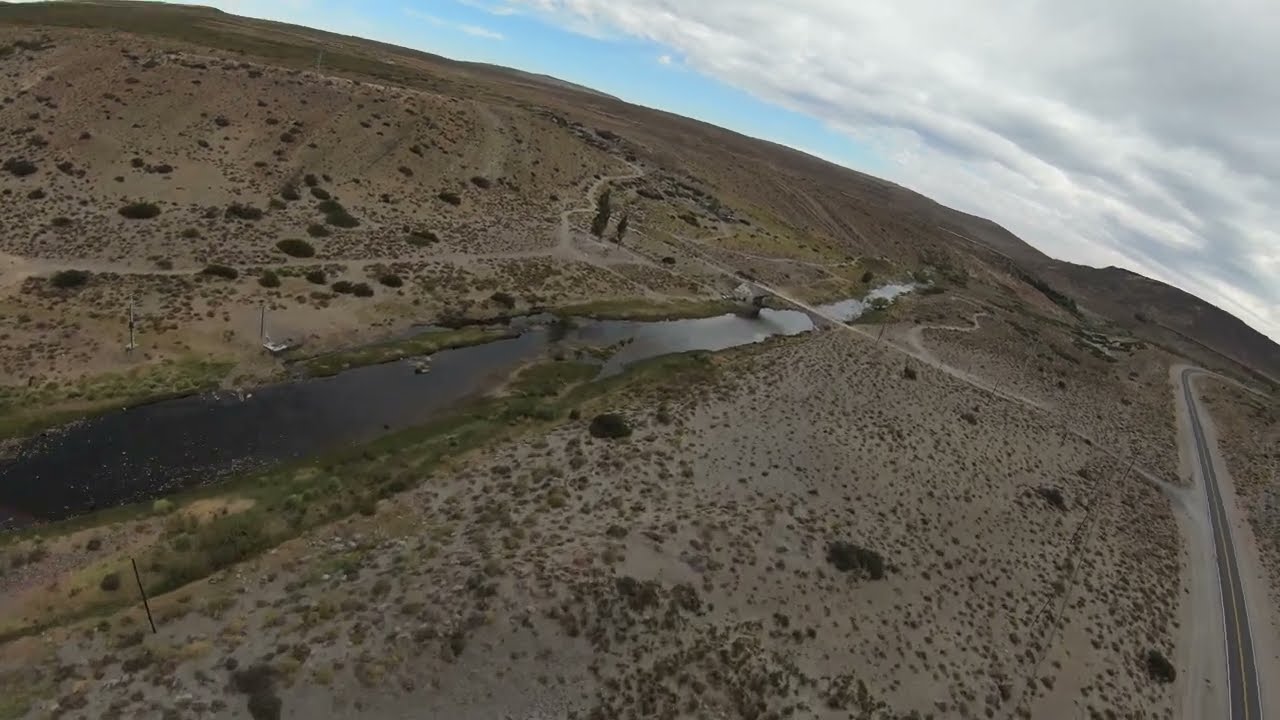This aerial drone shot captures a high-angle view of a rugged desert landscape. The ground is predominantly rocky and sandy with sparse, spotty shrub-like vegetation. Cutting through the arid terrain is a dark, narrow river or stream, flanked by slightly greener banks indicating a regular water presence. A small stone bridge crosses the river at the center of the image. 

To the right, a two-lane road with yellow markings extends towards the distant hills, curving sharply to the right as it nears the elevated terrain. A smaller, less well-paved road branches off to the left, leading to what appears to be farmhouses in the background. The image also features a small boat moored by the riverbank.

The sky above adds to the dramatic effect, with a patch of blue sky in the top left and dark gray to black storm clouds looming over the hills in the top right. The landscape is framed by mountain outlines in the far background, indicating a higher elevation despite the dominant desert environment.